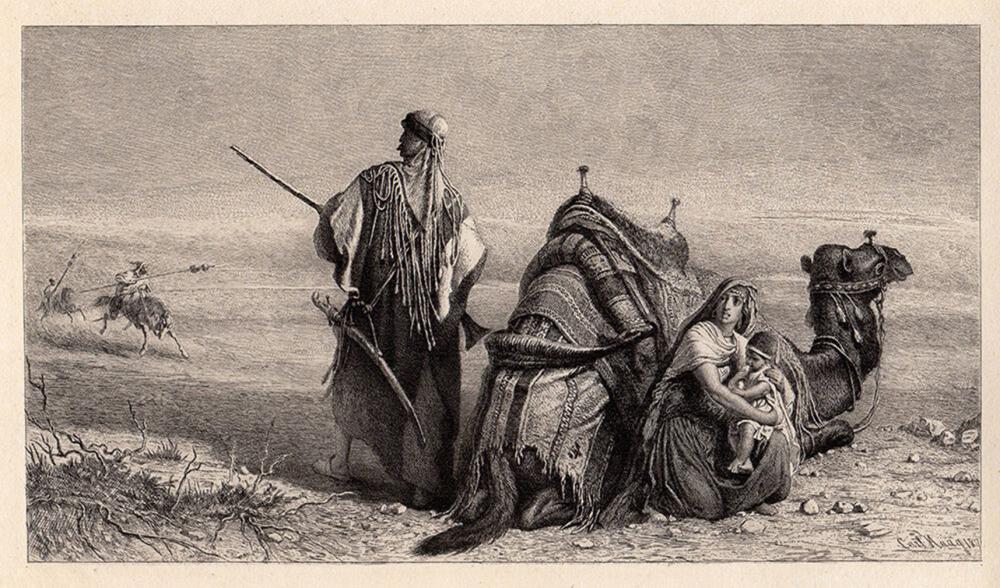This highly detailed black and white sketched illustration depicts an intense scene featuring an Arabian man, a woman, and a child with a large camel at the center. The camel, adorned with several layers of intricate fabrics, blankets, and rags, is lying down on its elbows and knees. The woman, dressed in a detailed wrap and dress, clutches her child protectively, using the camel for cover. To the left stands a man adorned in a scarf with tassels and carrying both a weapon and a sheathed sword, seemingly in a defensive stance. The scene is further heightened by two men on horses approaching from the background, their weapons drawn, as though they are charging at the family. The ground is rocky and cracked with rough brush visible in the foreground. An unreadable name is faintly inscribed in the bottom right corner of the image.